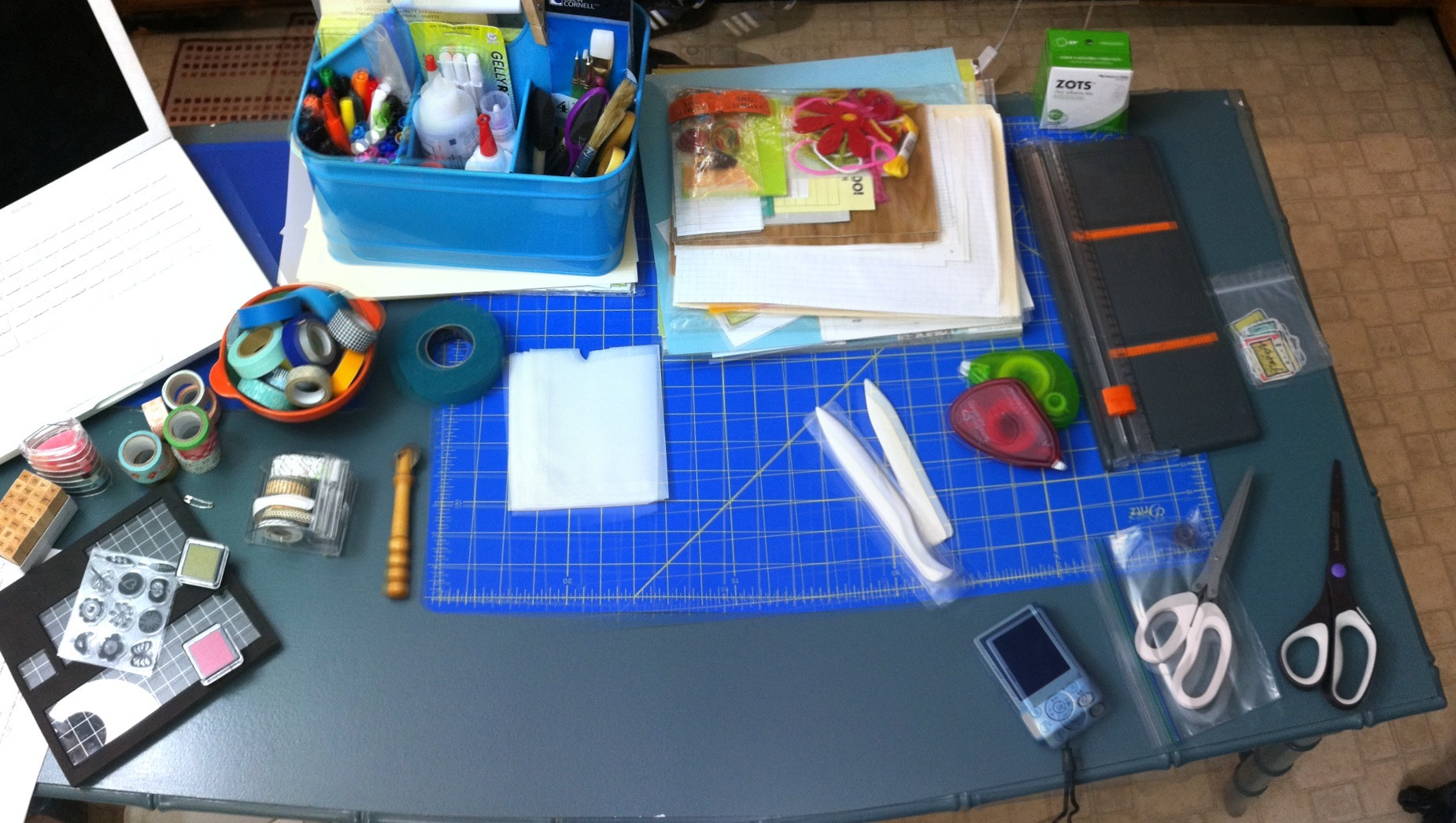This photograph captures a richly detailed workspace set against a backdrop of cream and brown tiled flooring. The focal point is a black table featuring an assortment of items neatly spread out. On the right side of the table, a pair of black scissors with white handle accents is placed next to another pair with white handles and silver blades, resting on a plastic surface. Adjacent to these is a digital camera.

To the far left, a collection of sewing supplies is visible, including spools of thread and a small black container with a clear cover. Nearby, an orange bowl containing tape adds a pop of color to the scene. Dominating the center of the workspace is a sizable blue piece of paper, patterned with white graph lines, along with additional white graph paper scattered around.

A blue bin holding markers and glue stands beside a sleek black paper cutter. The table also hosts an array of other graphing tools and supplies, indicating a meticulous, well-organized creative area.